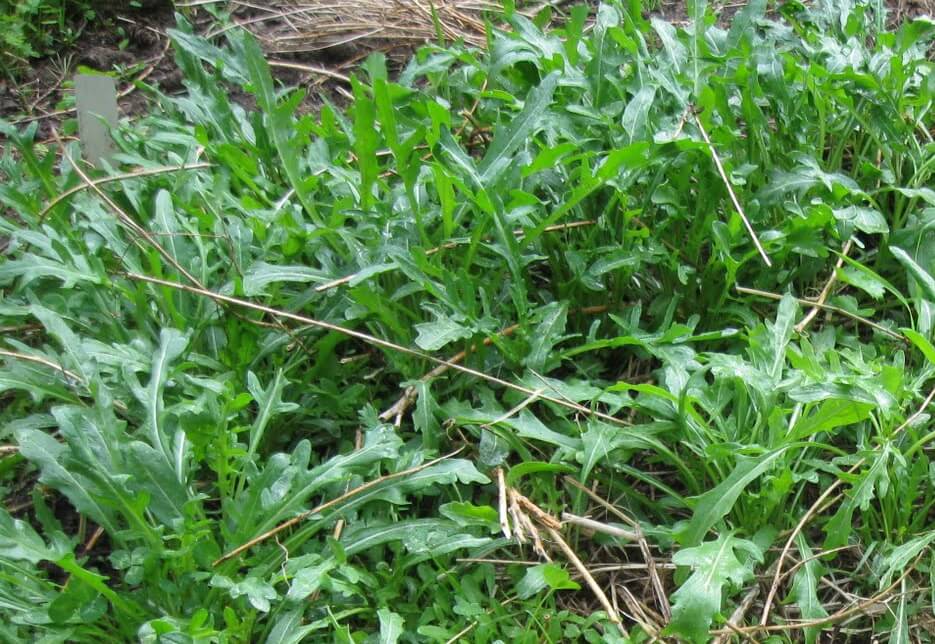This close-up outdoor photo captures a dense patch of greenery, likely a mix of leafy lettuce and various weeds, growing in a meadow or garden. The dark green leaves of the plants, which transition to a yellowish-green toward the center, are shown in rich detail. Interspersed among the foliage are dried stems, roots, and tan-colored dead grass, indicating a natural, somewhat unkempt setting. The foliage is so thick that it nearly obscures the dirt beneath, which peeks through sparsely. Thin, jagged-edged lettuce leaves and other types of broad and narrow weed blades are prominently visible, and the image is brightened by partial sunlight, suggesting an open and sunny environment. With no sky, sun, or clouds in view, the focus remains solely on the intricate and varied textures of the plant life below.